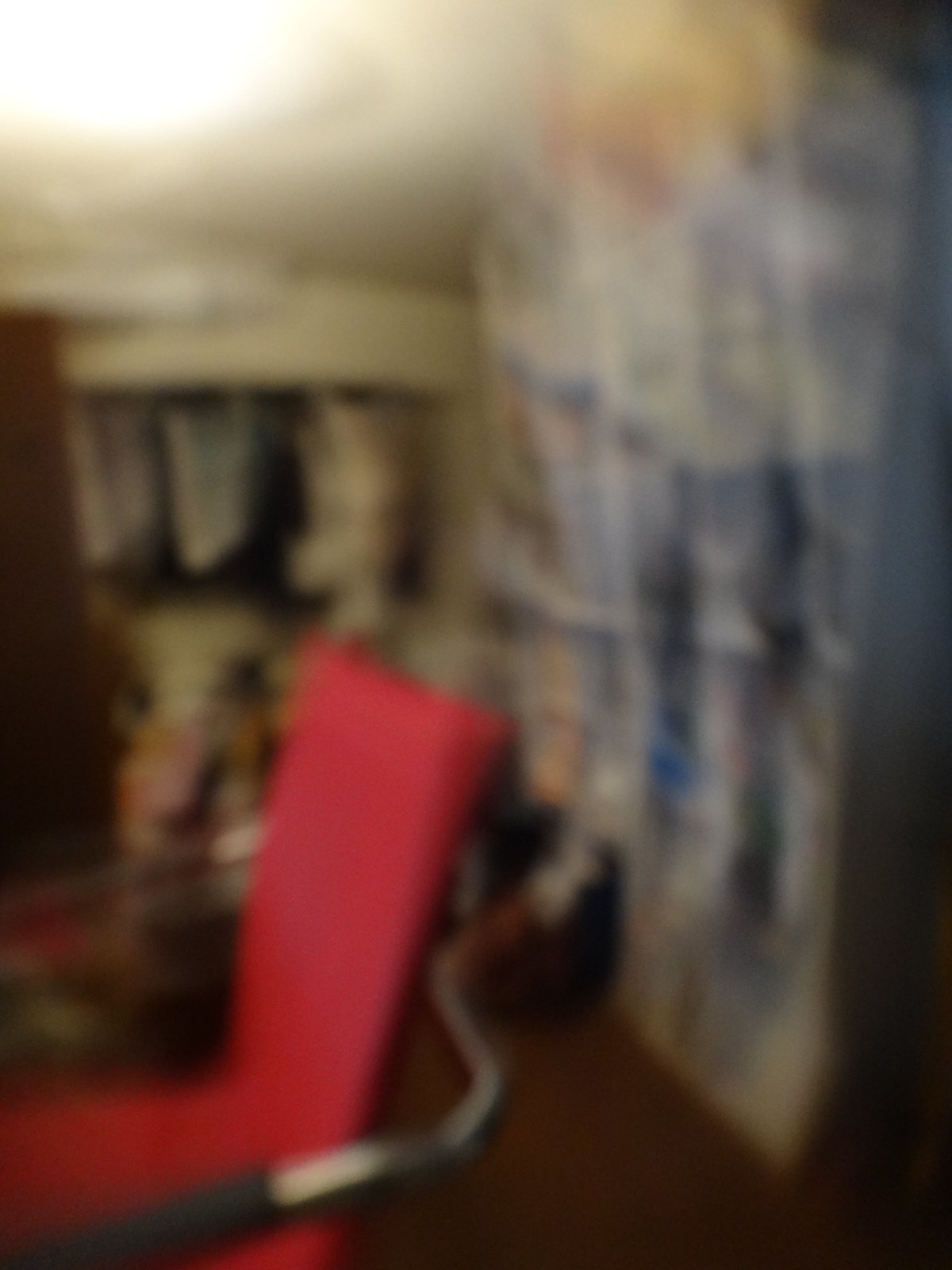This vertically-oriented, unfocused color photograph captures the interior of a room. Dominating the composition slightly below and to the left of the center is a red chair with a metal backing and side arms that end in black. The soft, blurred colors of the image include hues of yellow, white, black, and gray. To the right, there is a vague outline of a bookshelf. Above, a ceiling light occupies the top left corner. Various indistinguishable items are scattered along the back wall, their shapes and colors blending into the general softness of the background.